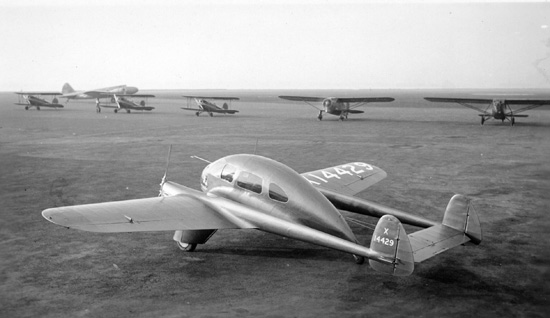This black and white photograph captures a historical scene of multiple vintage airplanes on a barren, dirt-covered airfield. At the forefront, a propeller plane from the World War I or II era stands out prominently. The plane, marked with the identifier "14-429" and an "X" on both its fuselage and right wing, features a distinctive bubble-shaped cockpit capable of seating 2 to 4 people. Its aerodynamic design includes a single propeller at the front, and a double tail fin with a horizontal spoiler connecting two vertical tubes extending from the wings. In the middle distance, five similar planes are lined up in a slightly diagonal formation, also facing the left. The background reveals a vast expanse of empty sky and distant land, emphasizing the isolation of this historic aviation scene.